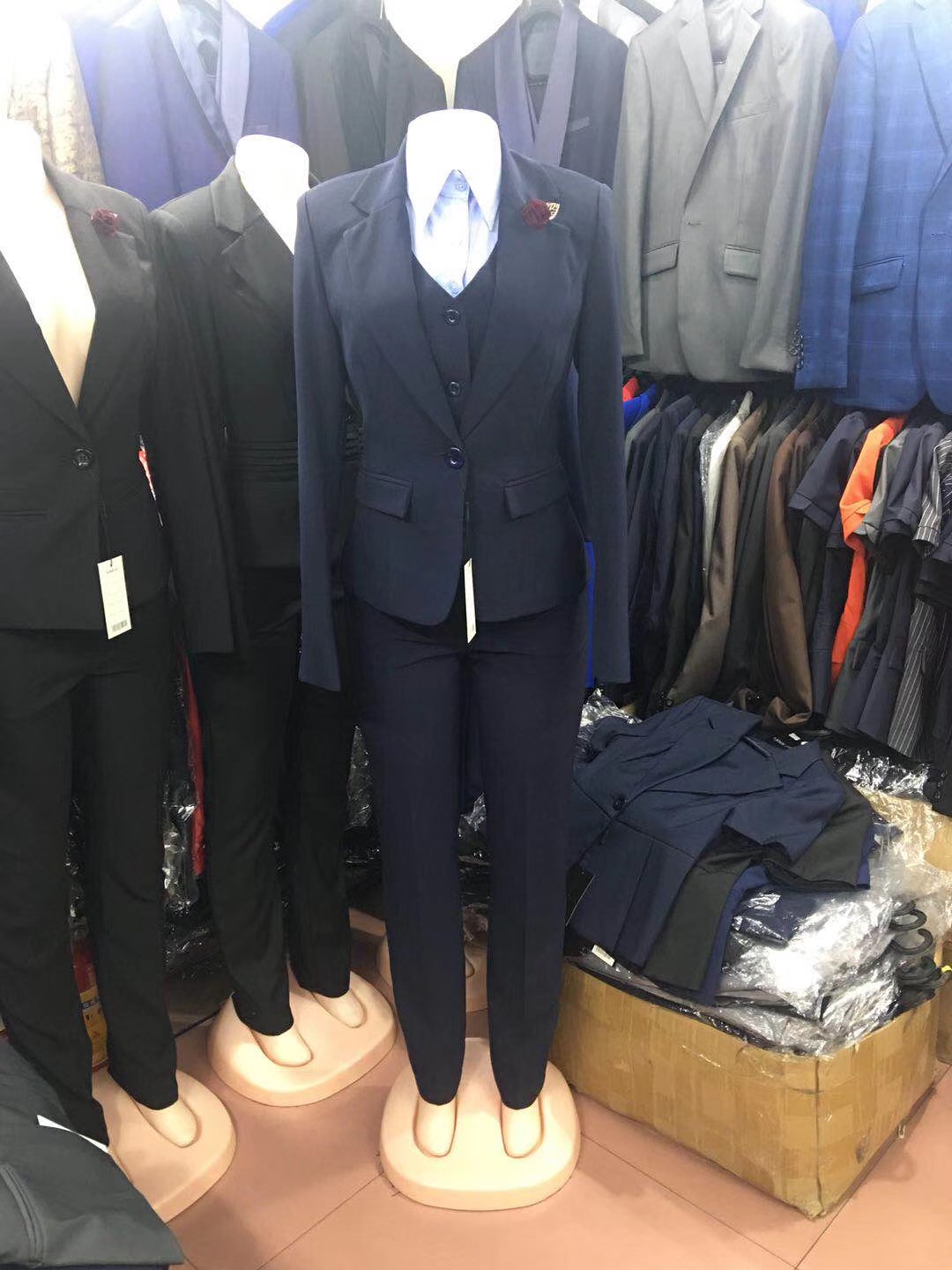The photograph captures a detailed view of a suit store. The floor, covered in peach-colored tiles, is scattered with items, including a cardboard box filled with various articles of clothing still in plastic packaging. Prominently to the left side and center of the image are three headless mannequins standing on small, wooden, round pedestals. Each mannequin is dressed in business attire. The central mannequin wears a dark navy three-piece suit, complete with a waistcoat, jacket, and trousers, and a faintly visible white shirt. A brown and white accessory, possibly a boutonniere or a handkerchief, adorns the lapel of the jacket. To the left of this mannequin stands another dressed in a black suit, while the third mannequin, positioned slightly behind and to the right, also sports a black suit. The display area behind the mannequins features a collection of various jackets and shirts hanging on racks. The edges of some t-shirt sleeves are barely visible beneath the jackets. In the lower left corner of the image lies a piece of greyish plastic, possibly a bag. A box filled with more clothing items not yet displayed sits in the lower right corner, with a navy blue jacket visible on top. The overall scene appears to be a well-stocked, albeit slightly cluttered, clothing store specializing in suits.